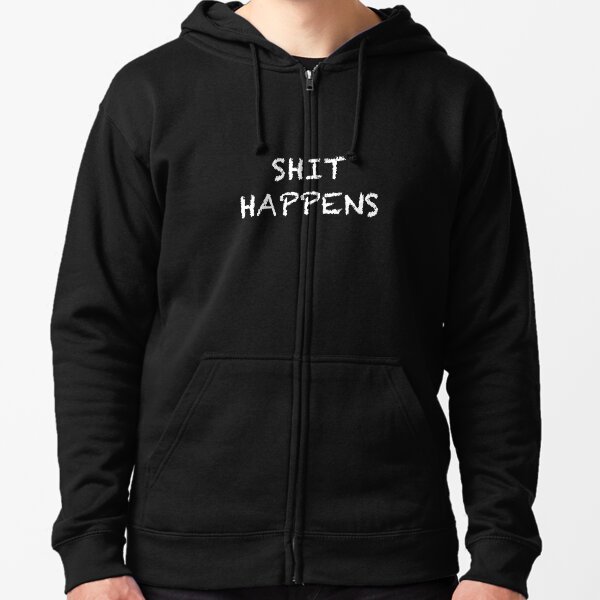The image depicts a person from just below the chin to the waist, against a white background. The individual is wearing a black hooded sweatshirt with a full front zipper, zipped up completely. The hoodie features two drawstrings hanging evenly down the chest, and the sleeves extend fully to the wrists with snug cuffs at the end. Only the proximal portions of the person’s hands are visible; no fingers are shown. The sweatshirt includes two front pockets with diagonal openings and an elastic cuff at the waist for a tighter fit. Written in uppercase white letters across the center of the chest are the words "Shit Happens." The visible portion of the neck highlights a prominent Adam's apple.